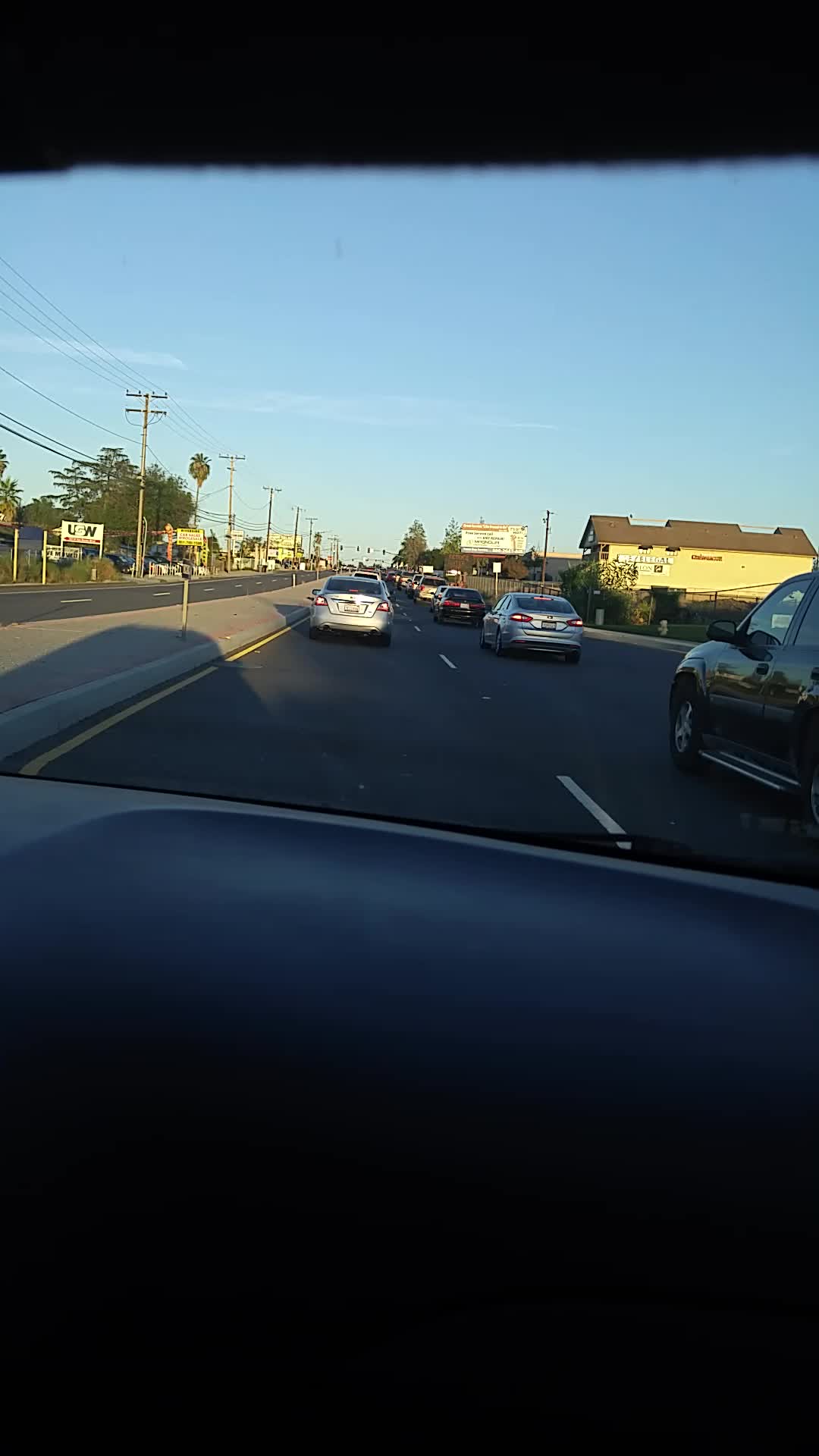A view from inside a car through the front windshield captures a bustling urban street scene. Ahead, two rows of cars are queued, all traveling in the same direction, with each vehicle spaced roughly 10 to 15 meters apart. Directly in front of the camera is a silver car. The sky overhead is a vibrant blue, adorned with a few light, wispy clouds drifting towards the left. To the right, a yellow building sits perpendicular to the road, indicating residential or commercial use. Electrical poles and various traffic signs line the streets, adding to the urban atmosphere. Another road runs parallel on the left, likely accommodating traffic in the opposite direction, though no vehicles are visible to confirm this. The overall scene captures the feel of a typical day on a busy city street, framed by clear skies and urban infrastructure.